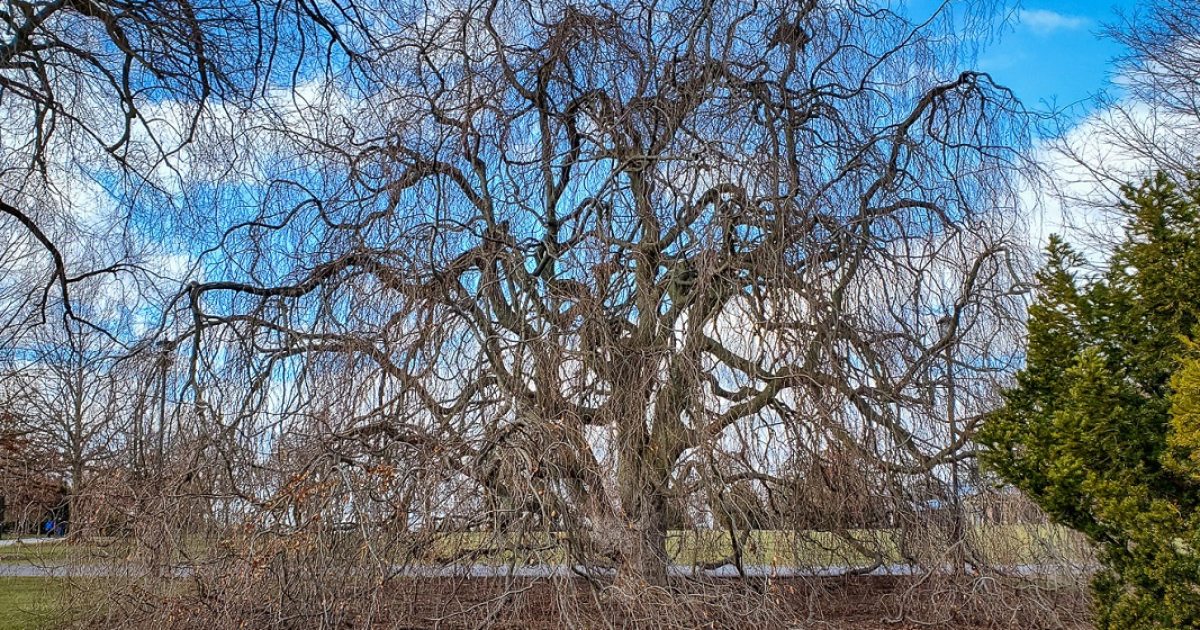The image captures a sprawling, older willow tree in a park-like setting, extending its long, leafless branches in every direction, some even touching the ground. Dominating the center of the landscape-oriented photo, this tree’s complex network of branches contrasts against a partly cloudy, light blue sky. Flanking the mighty willow are smaller green trees and bushes, creating a vivid scene of winter stillness with shades of green and brown. The ground beneath is a mix of grass, dirt, and mulch, with a visible gray pathway meandering from the lower left to the lower right. Streetlights with globe sections are dispersed throughout the background, adding to the ambiance of a public space, while hints of a road peek through the trees. The image's mid-day setting is indicated by the clear quality of the light.